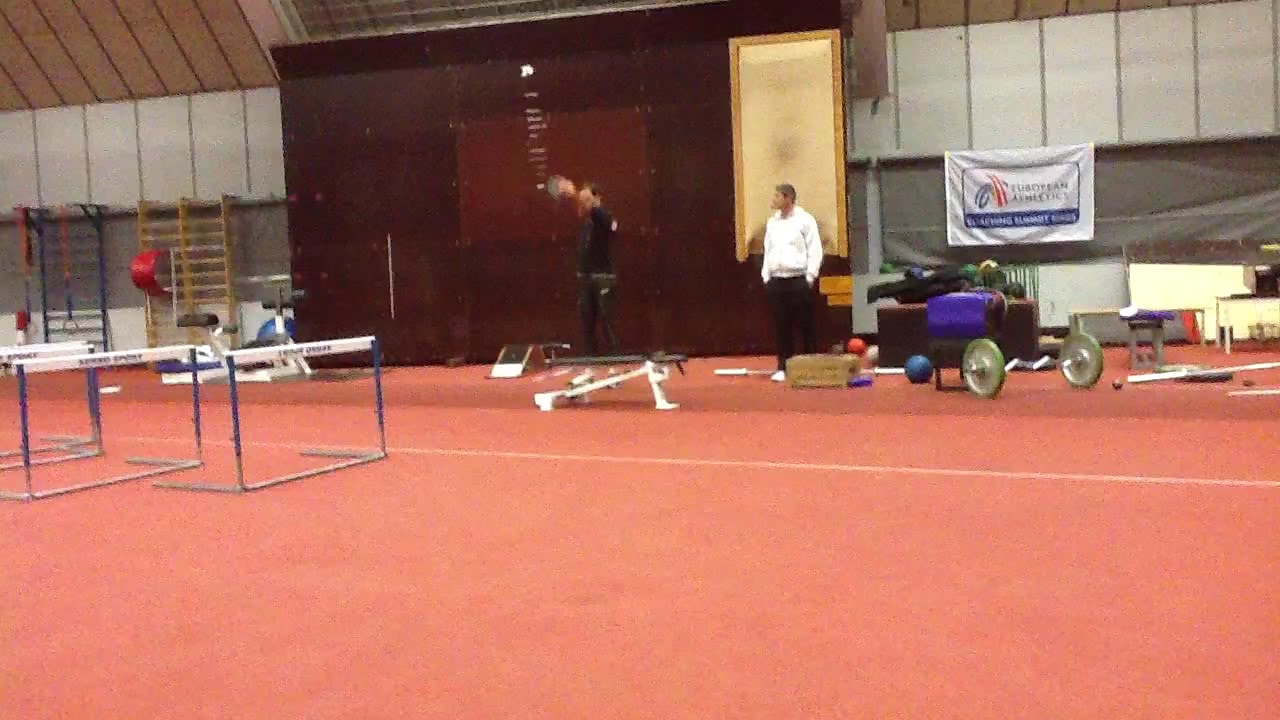The image depicts the interior of a sports gym or indoor track with a red floor scattered with various athletic equipment. In the foreground, on the left side, there are a set of hurdles used for jumping. The only visible person is a man wearing a white sweatshirt, black pants, and white sneakers. Positioned around him are a red ball, a blue ball, and a set of weights. To the left of the man is an unidentified white object, possibly gym equipment. The man stands behind a large black screen. In the background, a wooden sign with a brown finish can be seen, as well as a prominent long white wall with panels running the length of the image. The interior of a gabled roof is visible above. To the far right of the image, a white, red, and black sign with unreadable writing hangs. A left object is also hanging on the distant left wall. Various other gym equipment such as punching gloves, boxing gloves, smaller hurdles, and starter blocks are scattered around, emphasizing the gym's use for athletic training. Another man dressed in a black sweater and black pants can also be seen, standing nearby. Together, the scene appears to be set in a versatile space for athlete training and workouts.